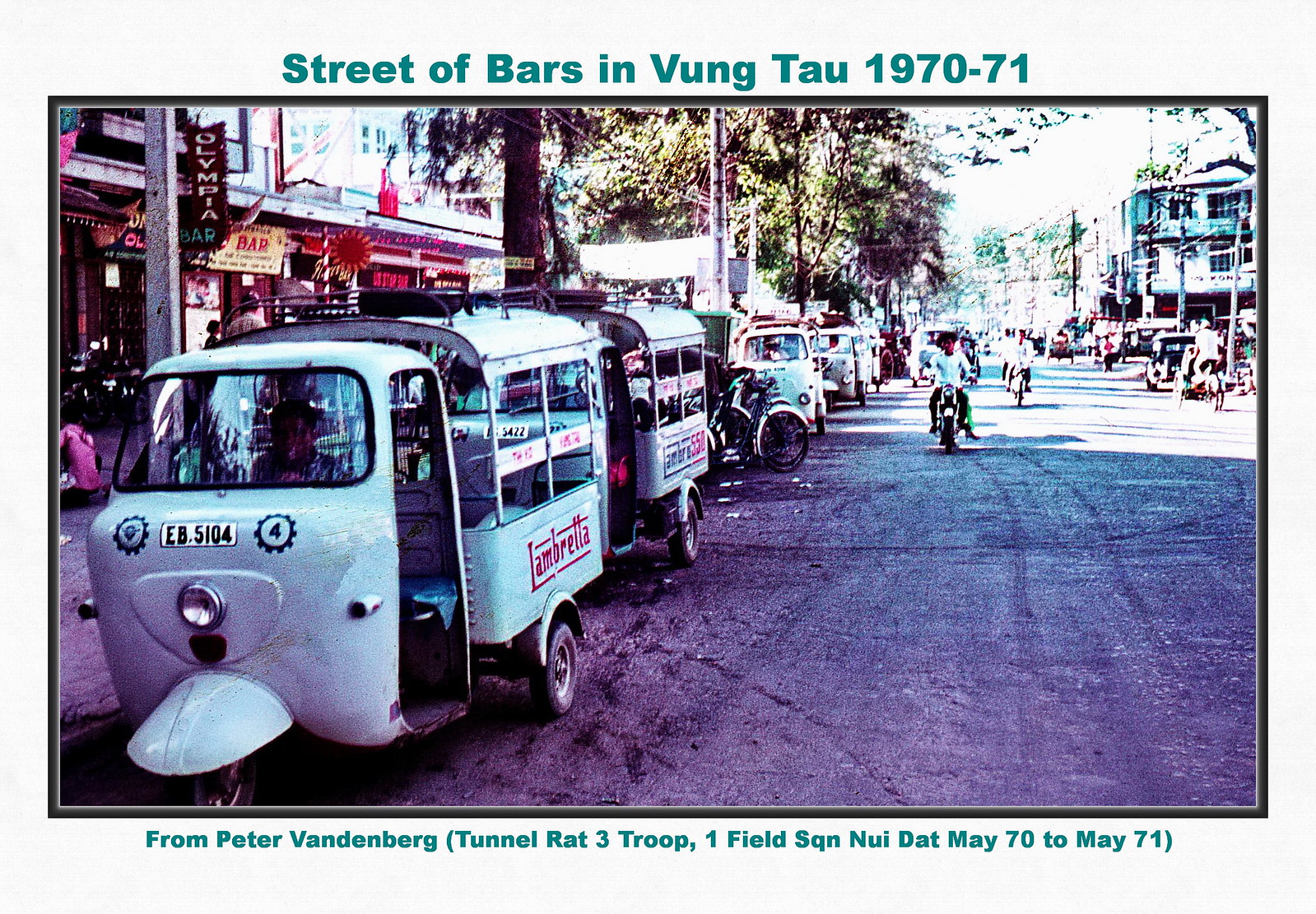A faded, full-color photograph captured by Peter Vandenberg in May 1970, titled "Street of Bars in Vung Tau, 1970-71," depicts a bustling street scene in Vietnam during the daytime. The image, labeled with Vandenberg's affiliation as part of Tunnel Rat 3 Troop, 1 Field Squadron, Nui Dat, showcases a vibrant street lined with bar establishments on the left side. A row of tuk-tuks, three-wheeled taxi-like vehicles popular in Asian countries, is parked along the sidewalk in front of these shops. On the opposite side, the street features numerous motorbikes ridden by locals. Trees and a building are visible in the upper right corner, adding depth to the outdoor setting. The perspective from the center of the street emphasizes the activity and atmosphere of this vivid moment in Vung Tau's history.